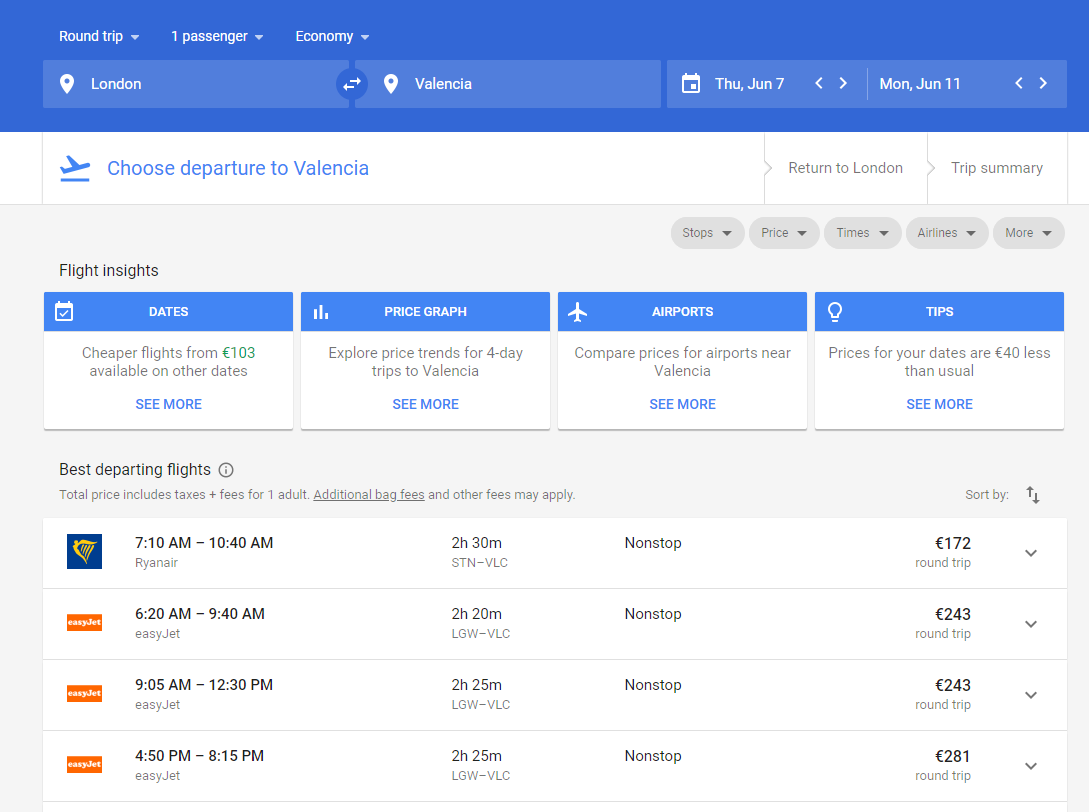This image is a detailed screenshot of a flight booking website, possibly for Summit Airlines or a flight comparison platform. At the top, round-trip tickets for a single passenger traveling in economy class are selected, with the journey originating in London and destined for Valencia. The travel dates are set from Thursday, June 7th to Monday, June 11th.

The section for choosing the departure flight to Valencia is currently highlighted. Subsequent steps would include selecting the return flight to London and reviewing the trip summary. The webpage header reads "Flight Insights," displaying various sections including:

- **Dates:** Indicates that cheaper flights starting at €103 are available on alternate dates.
- **Price Graph:** Offers an option to explore price trends for four-day trips to Valencia.
- **Airports:** Provides a comparison of prices for airports near Valencia.
- **Tips:** Notes that prices for the selected dates are €40 less than usual.

Each of these sections features clickable options for more details.

Below these sections, the "Best Departing Flights" are listed, with total prices including taxes and fees for one adult, while noting that additional baggage and other fees may apply. 

The flight options shown include:
1. A Ryanair flight departing at 7:10 AM and arriving at 10:40 AM.
2. An EasyJet flight departing at 6:20 AM and arriving at 9:40 AM.
3. Another EasyJet flight departing at 9:05 AM and arriving at 12:30 PM.
4. A final visible EasyJet flight departing at 4:50 PM and arriving at 8:15 PM.

The screenshot suggests there are additional flights available beyond what is visible in the image.